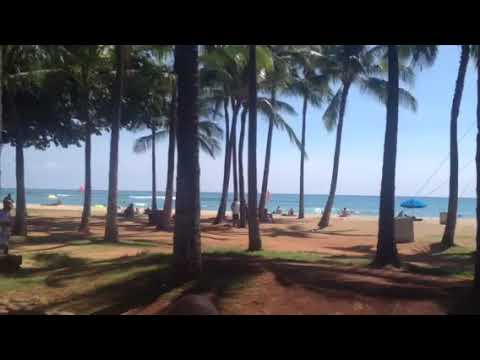The image captures a stunning tropical beach scene on a sunny day, with clear blue skies and calm waters. In the foreground, we're standing on a well-manicured grassy area interspersed with sandy dirt, surrounded by a dense cluster of tall palm trees that create a canopy of shade. The palm trees extend from the grassy area towards the sandy beach, where they continue to grow. Around us, several people are present; some are walking, some are standing, and others are seated closer to the water, enjoying the serene environment. A noticeable feature is a blue-topped umbrella on the right side, providing a shaded area where people are relaxing. Off in the distance, the beach transitions smoothly into the clear, blue ocean. Additional details include a possible sighting of a wakeboarder or people on boats far out at sea, suggesting recreational activities. This picturesque setting hints at being near a hotel or a public access area, adding to the inviting and potentially communal atmosphere.